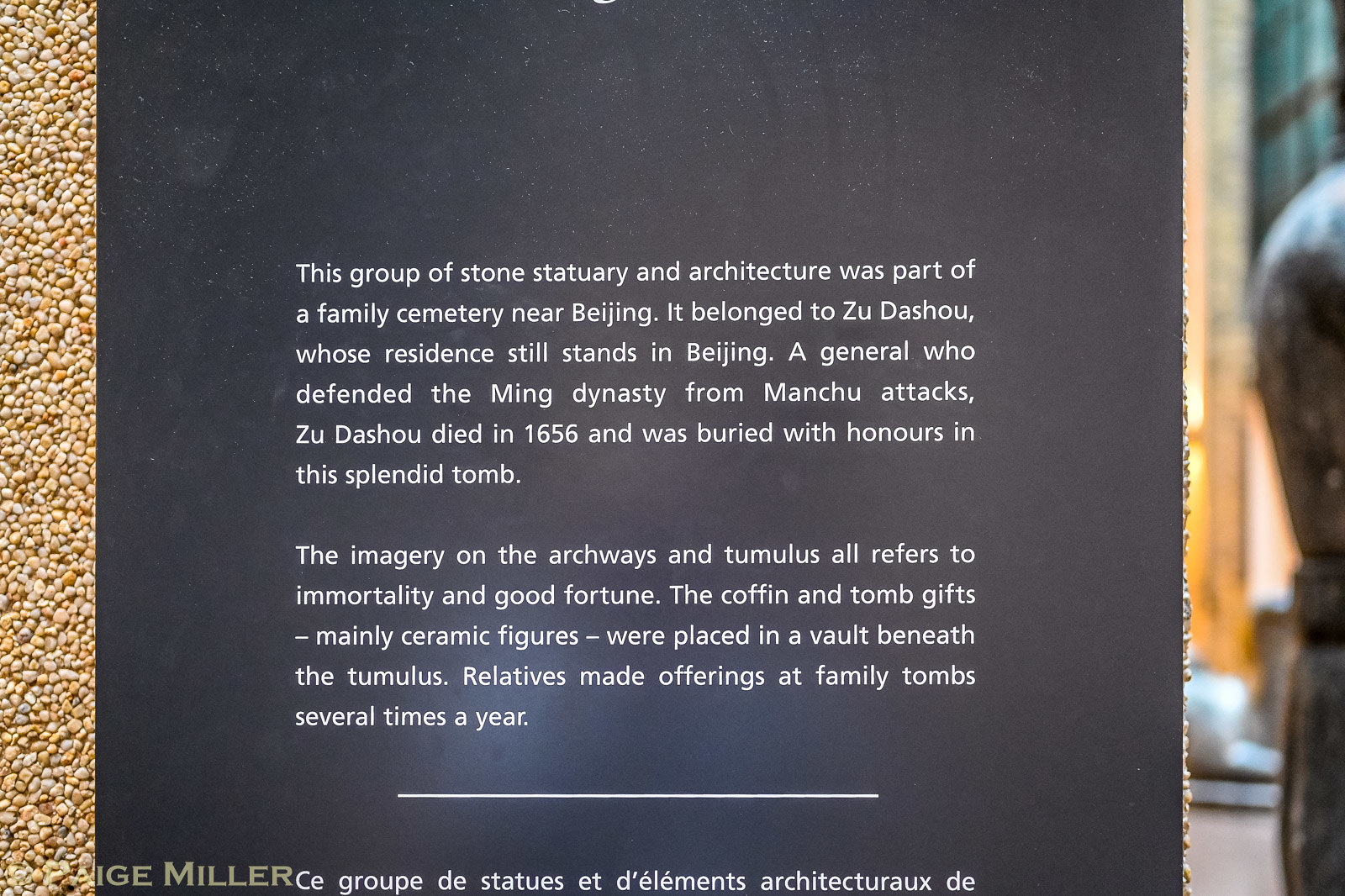This image shows a black plaque mounted on a stone wall that appears to be composed of small pebbles. The plaque, featuring white text, is situated on the side of a building in an outdoor setting. To the right, partially visible, is the back of a statue and what seems to be an indoor area, possibly an office or building lobby. The text on the plaque commemorates a group of stone statuary and architecture that belonged to a family cemetery near Beijing. This cemetery, including this splendid tomb, was dedicated to General Zhu Dashu, who defended the Ming Dynasty from Manchu attacks and died in 1656. The elaborate imagery on the archways and tumulus symbolizes immortality and good fortune. Beneath the tomb lies a vault where the coffin and numerous ceramic figures, meant as tomb gifts, were placed. Family members traditionally made offerings at the tomb several times a year. Below the main inscription, there is a line followed by similar text in French, indicating a bilingual commemoration.